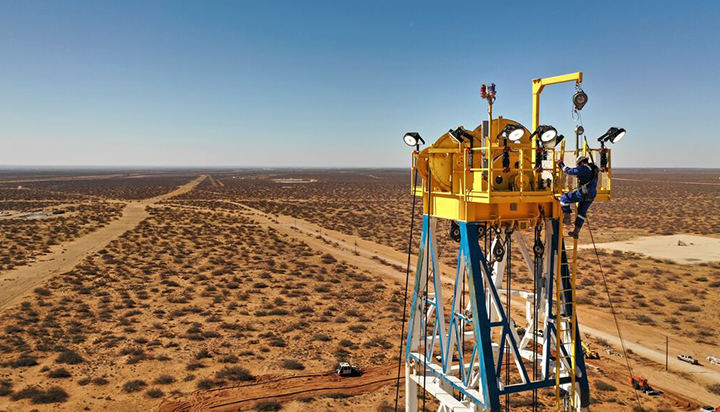This expansive image captures a flat, wide-open desert landscape, stretching out without any hills, under a clear blue sky occupying the upper third of the frame. The vast expanse of sandy brown dirt below is punctuated with sparse shrubs and crisscrossed by two prominent dirt roads: one originates in the lower right corner and extends diagonally into the distance, intersecting with another road that angles away from the lower left side. Adjacent to these roads lies a flat, cemented area towards the center-right of the image.

Dominating the foreground is a tall tower, presumably part of an oil exploration or drilling rig, with its base out of view. The structure features a mix of white and blue metal support poles, while its upper portion is painted yellow and equipped with numerous angled lights. At the top, there is a yellow housing with circular winches and wires, and a potential weighing scale extension.

Climbing up a yellow ladder affixed to the tower is a man dressed in a blue uniform, brown boots, and a safety helmet. He is secured with a safety belt and pulley system to prevent falls. Below the tower, intermittently visible vehicles - including cars and tractors - traverse the dirt roads, contributing to the sense of scale and activity within this desert setting.